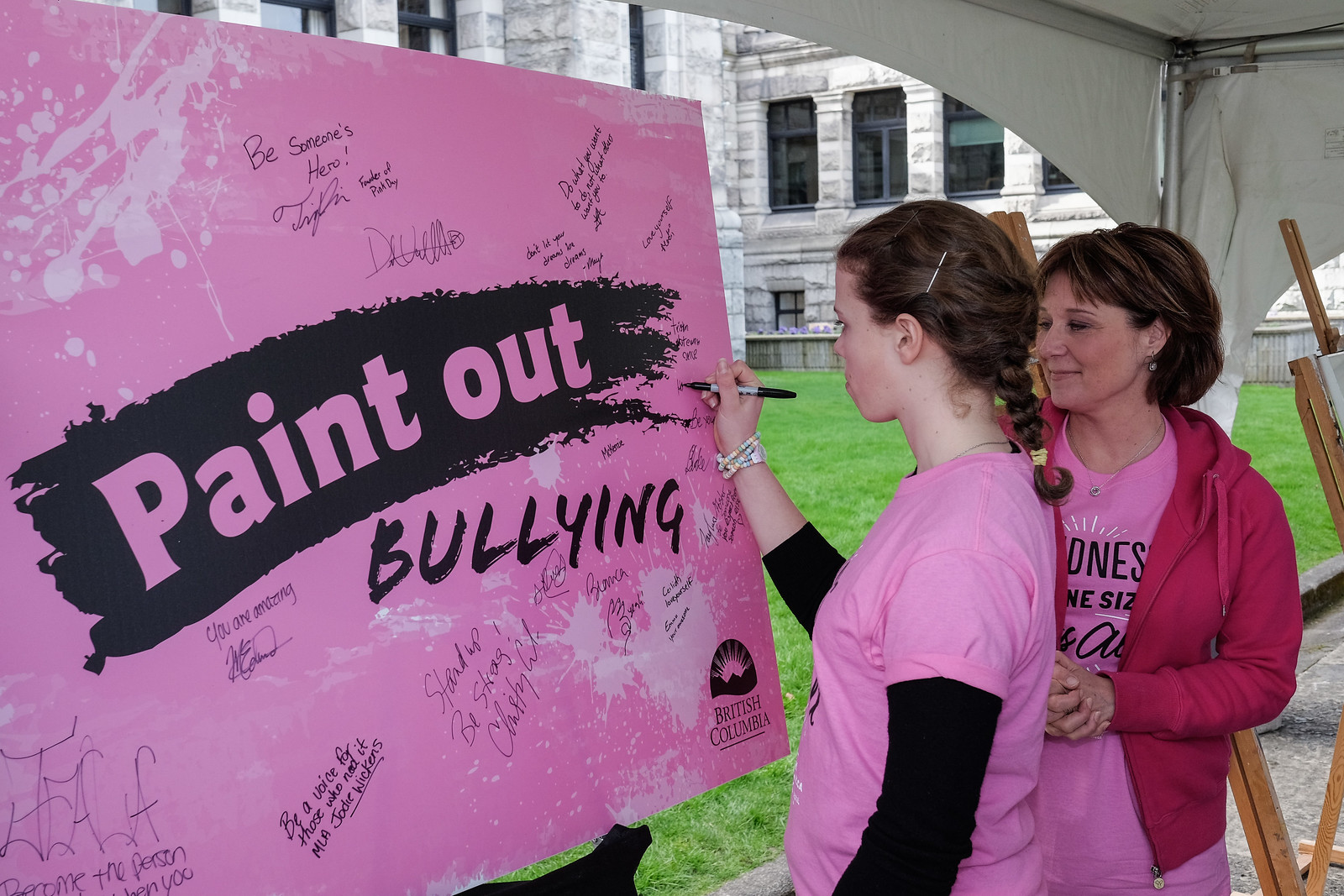In this vibrant outdoor scene, a young girl with brown braided hair, adorned with two pins, diligently writes with a Sharpie on a large pink board that prominently displays the text "Paint Out Bullying" in bold black and pink letters. The board, filled with inspirational messages and signatures like "Be someone's hero" and "Don't let your dreams be dreams," is part of an anti-bullying campaign, seemingly led by the school, as indicated by the inscription "British Columbia" at the bottom. The girl, wearing a pink shirt over a black long sleeve, and colorful bracelets on her wrist, adds her contribution to the collective message of encouragement. Standing next to her is a smiling woman with short brown hair, wearing a pink shirt similar to the girl's, a pink hoodie, a necklace, and an earring, with her hands clasped together. They are positioned under a large gray canopy with a backdrop of green grass and a gray building, suggesting a school or community setting where many have gathered to support this cause.